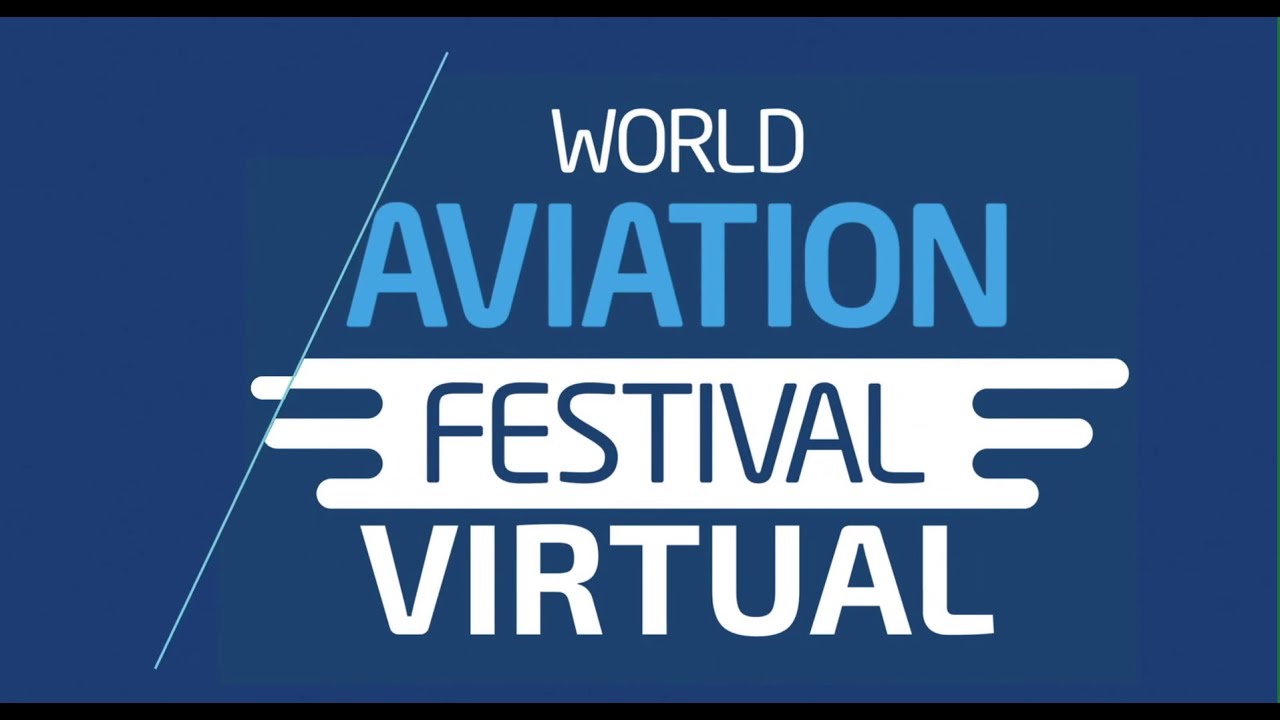The image features a horizontally aligned rectangular graphic with a navy blue background, flanked by black borders at the top and bottom. Centralized text in all capital letters reads: "WORLD" in white, "AVIATION" in light blue, "FESTIVAL" in dark blue on a white background with jagged edges, and "VIRTUAL" in bold white. A thin, slanted light blue line runs from the bottom left to the top right, intersecting with the words "AVIATION" and "FESTIVAL." Additionally, three white lines extend horizontally from the sides of the word "FESTIVAL".